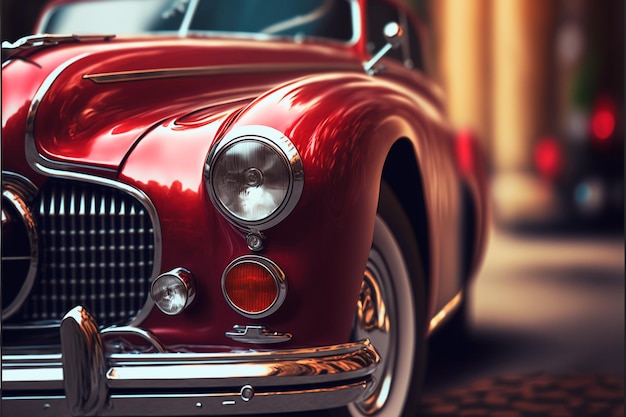This photo captures a vibrant red, vintage luxury car from a close-up angle, focusing primarily on the front left side. The image highlights the car's intricate design characteristics, including its substantial chrome bumper, prominent round headlights, and distinctive curves around the hood and above the wheel. The front left tire, featuring a classic white sidewall, is the most prominent part of the vehicle in the shot. The background is intentionally blurred, possibly including a street scene with indistinct columns and a red light, drawing all attention to the car’s striking details. The overall styling suggests the car dates back to the 1940s or early 1950s, reminiscent of those seen in places like Cuba today. The image is highly stylized, adding to its timeless appeal.